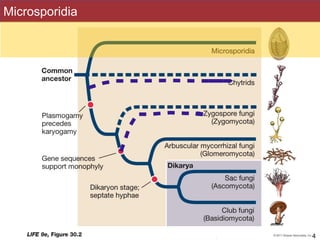The image depicts a detailed flowchart titled "Microsporidia," featuring a horizontal diagram illustrating the evolutionary development and connections between different fungi. At the top, there is a red bar with the title "Microsporidia" in white font, followed by a yellow bar and a light peach-colored rectangle containing various lines that connect to both the right and left columns of the chart. The right column features descriptors and icons for each respective line. Heading down the right side vertically are images of fungi, such as mushrooms, and text describing different stages and relationships. Key terms include "common ancestor," "Plasmogamy precedes Karyogamy," "gene sequences support Monophyllae," and classifications like "Sac Fungi (Ascomycota)" and "Club Fungi (Basidiomycota)." The diagram is characterized by its multiple colors, including red, yellow, purple, green, bluish-green, tan, white, and black, and appears to be sourced from a science textbook focusing on fungal biology. The specific diagram is labeled Figure 30.2.